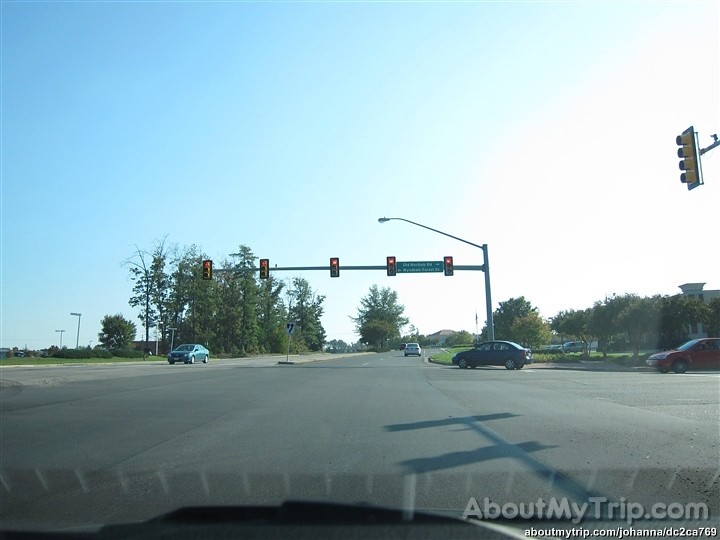A photo captured from inside a car through the front windshield at an intersection. The bottom right corner displays the watermark "aboutmytrip.com." The traffic light is red for the lane in which the car is positioned. There are five red lights visible: two for turning and three for going straight. The intersection consists of two lanes. In the right-hand lane, a small, darker-colored car is preparing to move forward, with a red car positioned directly behind it. On the left-hand lane for oncoming traffic, there's a solitary blue car. The left side of the road lacks any visible buildings or structures, while the right side features a cluster of trees and a building.